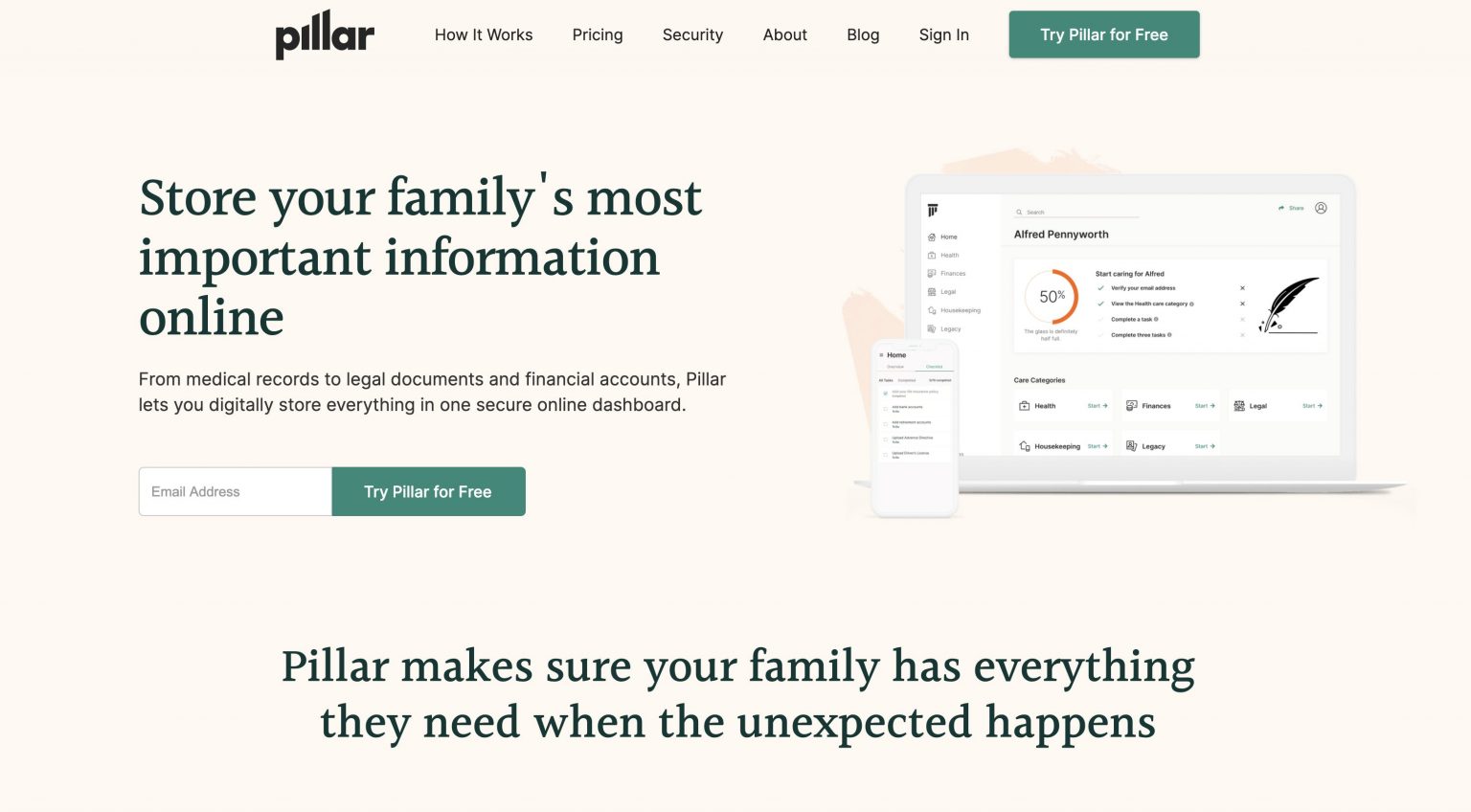This image depicts the homepage of "Pillar," a web service designed to store and manage your family's essential information securely online. The page features several navigation tabs, including "How It Works," "Pricing," "Security," "About," "Blog," and "Sign In." Prominently displayed is a green "Try Pillar for Free" button. The background of the page has a soft peach hue, creating a warm and inviting atmosphere.

In large green text, the headline states, "Store your family's most important information online," followed by detailed black text explaining the service: "From medical records to legal documents to financial accounts, Pillar lets you digitally store everything in one secure online dashboard." Below this description is a white input box for entering an email address, accompanied by another green "Try Pillar for Free" button.

To the right side of the screen, there's an image of a white laptop with a smartphone leaning against it, both featuring displays that aren't clearly readable. Underneath this visual, additional green text reads, "Pillar makes sure your family has everything they need when the unexpected happens," emphasizing the platform's value and purpose.